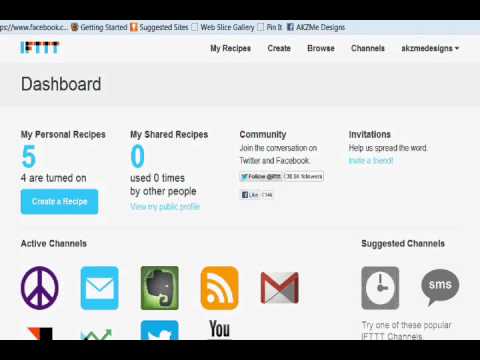A blurry and pixelated screenshot of a desktop displaying the IFTTT Dashboard. The image has a squished aspect ratio with black bars at the top and bottom. In the top left corner, "IFTTT Dashboard" is prominently displayed. To the right, there are several clickable text links in black, including "My Recipes," "Create," "Browse," "Channels," and a drop-down menu labeled "Designs."

Below this navigation bar, the dashboard features "My Personal Recipes" with a large blue number "5," indicating five recipes, four of which are currently active. "My Shared Recipes" shows a big blue "0," reflecting zero recipes used by other people.

Further down, under the "Community" section, users are encouraged to join the conversation on Twitter and Facebook, with options to share on these platforms. The "Invitations" section is also noted.

At the bottom, under "Active Channels," various icons are displayed, including an RSS feed, Gmail, Twitter, and YouTube, representing the user's connected services.